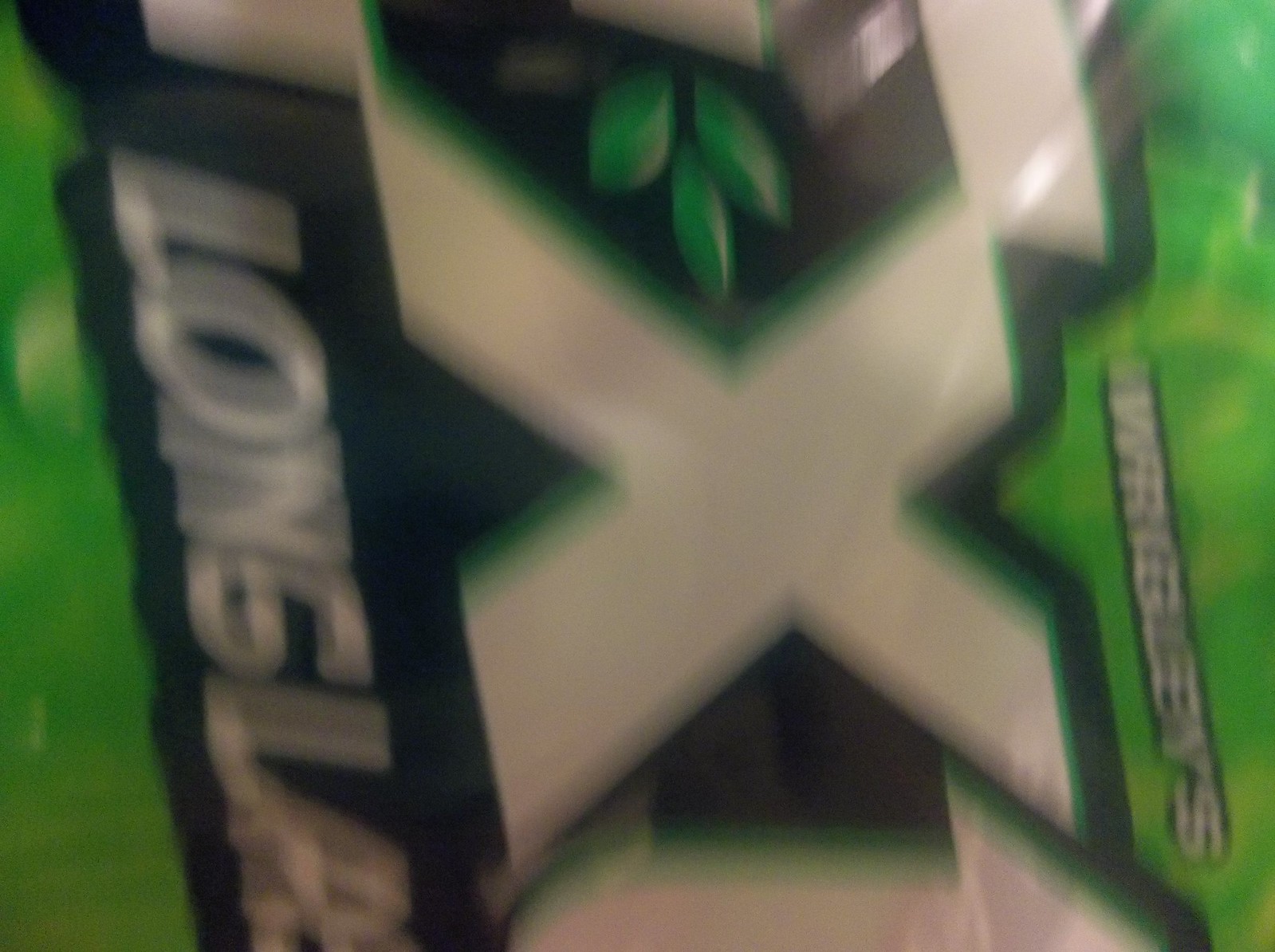A highly magnified image showcases a plastic food packet. The packet, oriented at a 90-degree angle to the right, features a prominent green color on both the far right and far left edges. To view the image correctly, one would need to rotate their head 90 degrees to the right. The focal point of the image is a close-up of some text on the packet. On the far right, the word "Wrigley's" appears, albeit blurred and distorted. Below this, large, bold, 3D letters with black borders spell out "E, X, T." Further down, in a similar bold, capitalized, 3D style with black borders, is the partial word "LONSLA," trailing off out of the frame. A light source situated at the top right corner casts a reflection and glare on the packaging, adding to the complexity of the image.